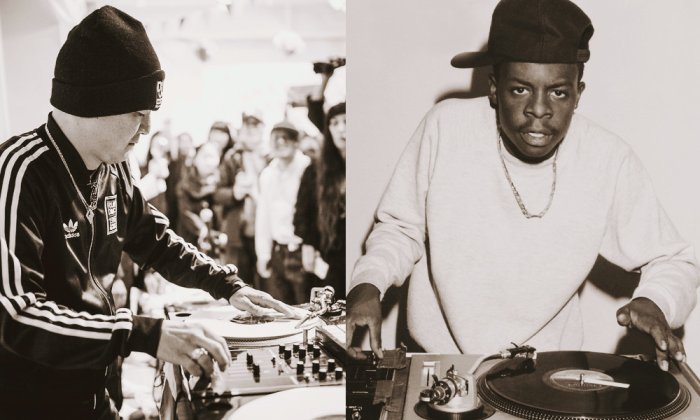This is a composite black-and-white image featuring two vintage DJs and their turntables. The left image captures a side profile of an Oriental man in an Adidas tracksuit and a black beanie hat. He is engaged in DJing, with one hand on the turntable, scratching records, and the other hand adjusting the dials on a mixing pad adorned with black knobs. The background includes a crowd, some holding up their phones, intently watching the DJ perform. The right image showcases a black man wearing a white long-sleeved sweatshirt, a thin gold necklace, and a black baseball cap turned to the side. He is looking directly at the camera with his hand poised over a turntable, appearing ready to make DJ scratch sounds. Both images evoke a nostalgic ambiance and highlight the classic art of DJing.